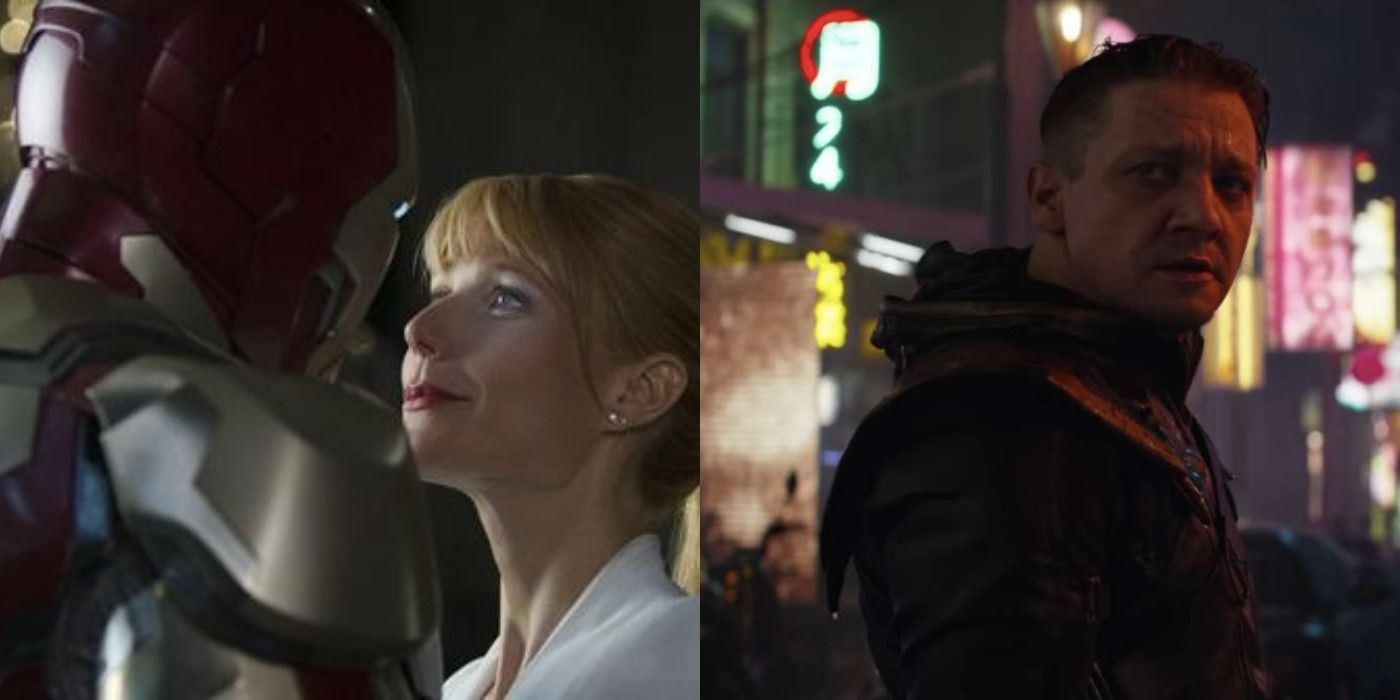This image features a split-screen thumbnail from a YouTube video, themed around the Marvel Cinematic Universe, specifically "Avengers: Endgame" and "Iron Man 3." On the left, from "Iron Man 3", we see a poignant scene with Pepper Potts, portrayed by Gwyneth Paltrow, donning a white blouse and red lipstick, her red hair tied back into a bun. She gazes intently at the red and gold Iron Man armor, which has a transparent faceplate revealing a man inside, suggesting an emotional moment of connection. On the right, a still from "Avengers: Endgame" shows Clint Barton, also known as Hawkeye or Ronan, played by Jeremy Renner, standing in a vibrant urban setting adorned with blurred neon signs, notably in Japan. He wears a dark leather armor with gold accents and a hood draped behind his head, exuding a brooding presence likely after exacting revenge for his family’s demise during Thanos’s snap. The composition suggests a narrative contrast between serene contemplation and intense aftermath.